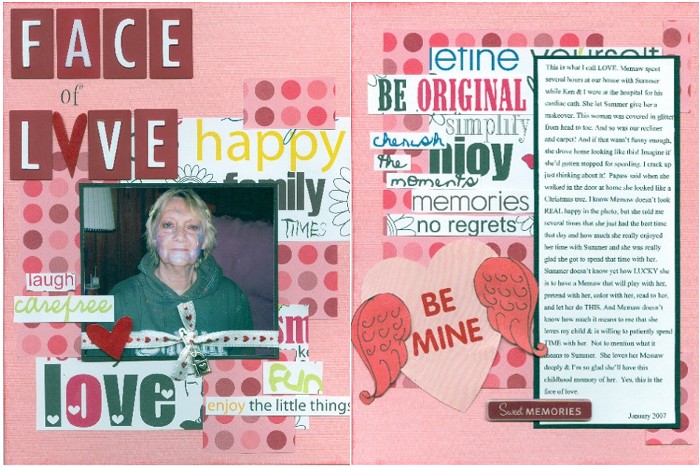The image is a landscape-oriented color photograph of an open two-page collage, with both pages featuring a pink paper background. The left page is topped with red rectangular panels, each containing a white letter, spelling out "face of love" with the 'O' creatively replaced by a dark V in hand lettering. Below this title is a color photograph of a woman in her 40s or 50s, wearing a green hoodie and smiling upwards at the viewer. The photograph is adorned with a white ribbon featuring a heart motif. Surrounding this central image are various words and phrases, such as "happy family times," "laugh," "carefree," and "enjoy the little things," crafted from cut-out letters and designs.

On the right page, the collage continues with cut-out words in diverse fonts and styles, including "define," "be original," "simplify," "cherish," "joy," "memories," and "no regrets." A prominent feature on this page is a pink Valentine heart with the phrase "be mine" and pink angel wings. Additionally, there's a vertical column of black text on a white background, though it is too blurry to be read clearly. A message, "save memories," and the date "January 2007" appear at the bottom right corner. The design of the entire spread is a playful and heartfelt scrapbook style, simulating a child's book with a melange of various images and textual elements, creating an affectionate and nostalgic scene.